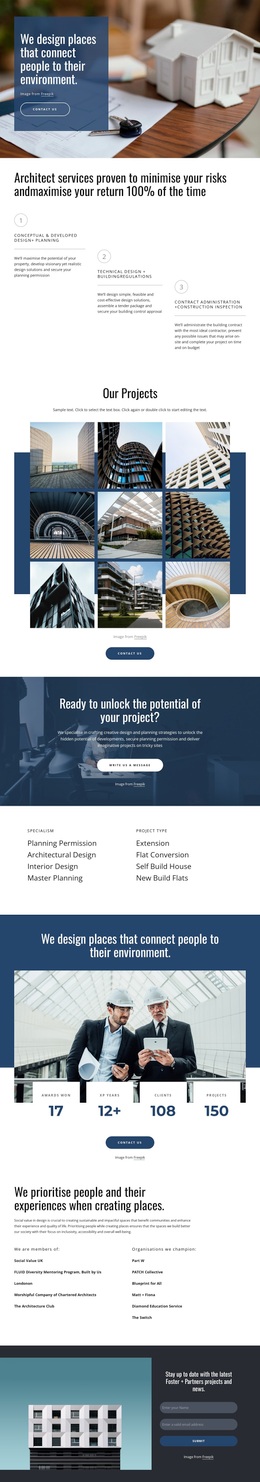The image depicts a detailed website template designed for a corporate and industrial business focused on architecture and design services. The webpage layout is vertically extensive, encompassing five main sections stacked one above the other, resulting in a very long vertical image that makes finer text difficult to discern.

At the top, the homepage features a prominent picture banner displaying a round table set up for a meeting. Scattered across the table are various forms, contract papers, a set of keys, and a small 3D model of a house. Overlaid on the banner image is a headline that reads: "We design places that connect people to their environments."

Below this visual, there is a section of large, easily readable text promoting the company's architecture services. The text asserts, "Architect services proven to minimize your risks and maximize your return 100% of the time."

Further down the page, there are additional text segments and several high-resolution stock images showcasing intricately designed tall buildings and complex architectural structures. One notable tagline declares, "Ready to unlock the potential of your project?" echoing their core message of creating connective and environment-integrative designs.